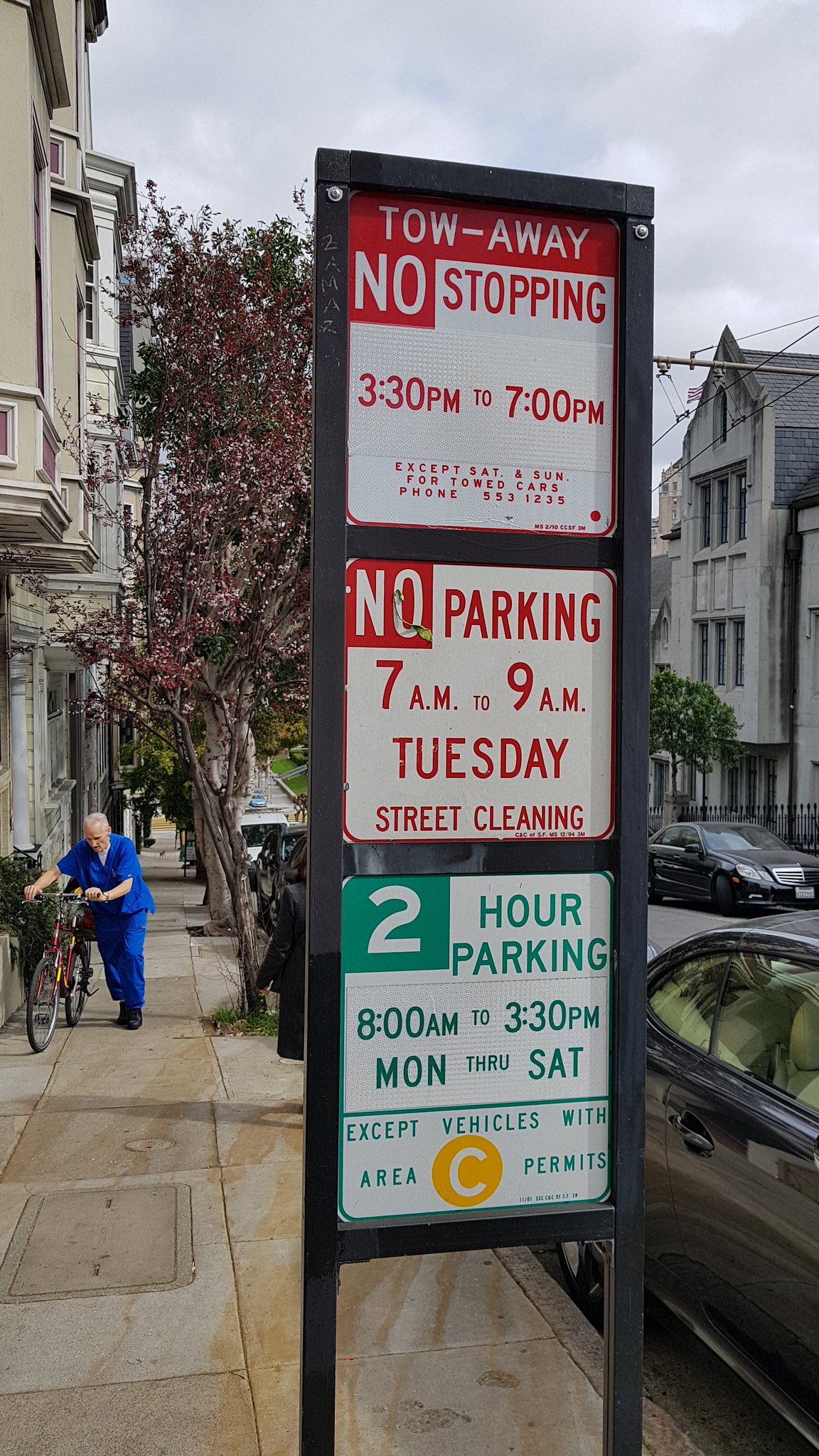This image depicts a typical bustling neighborhood street in a U.S. city, most likely San Francisco or Boston, identified by the trolleybus wires overhead. Central to the photo is a stacked set of parking restriction signs on a sidewalk, detailing: "Tow Away, No Stopping, 3.30 PM - 7 PM, Except Saturday and Sunday," "No Parking, 7 AM - 9 AM, Tuesday, Street Cleaning," and "Two Hour Parking, 8 AM - 3.30 PM, Monday through Saturday, Except Vehicles with Area C Permits." An older man, possibly a healthcare worker, dressed in bright blue pants and a shirt, can be seen in the background, pushing a bicycle up the street. To the left, a parked Mercedes is visible alongside a vibrant green and red tree, while a row of other parked cars lines the right side of the street, all bathed in daylight.